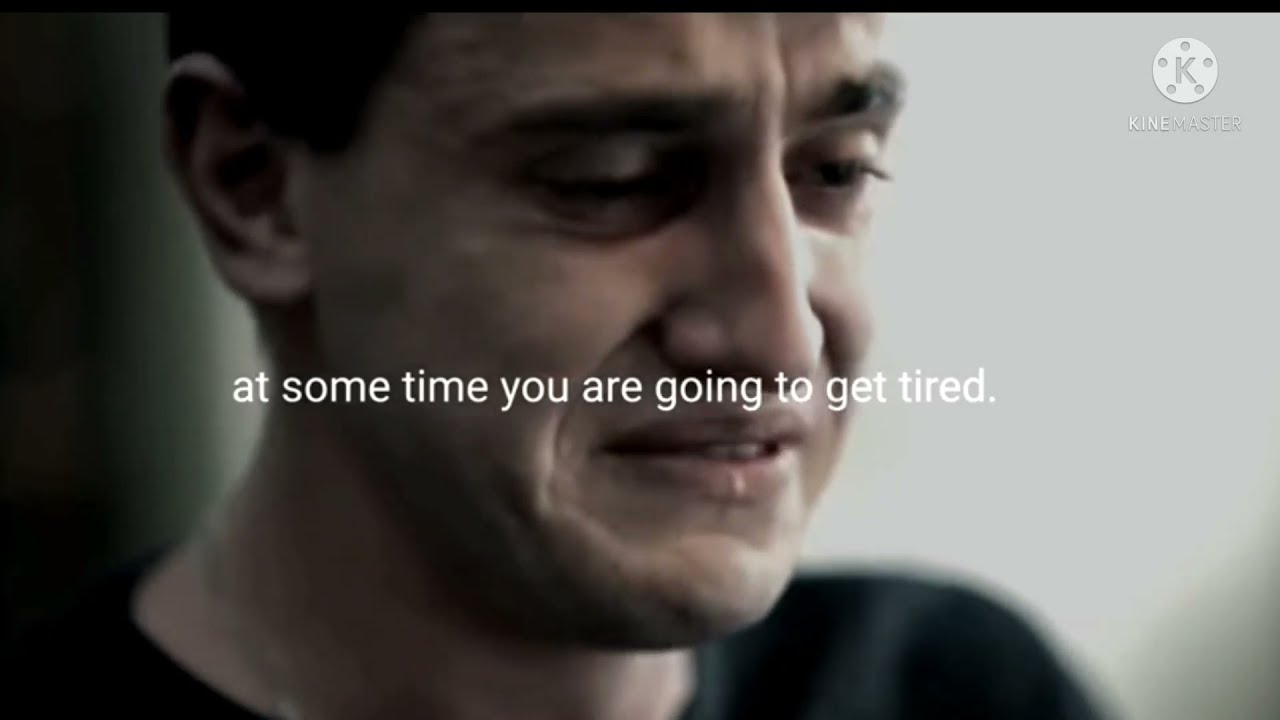The image appears to be a screenshot of a video, likely from a movie, show, or commercial. It features a Caucasian man with short brown hair, possibly in his 40s, who looks like he is on the verge of crying. He is wearing a black shirt, though parts of his attire and the background are somewhat blurred. The man is seemingly in a room with white walls and is sitting down, potentially in a waiting area with other people, as suggested by a blurry shoulder next to him. In the middle of the screenshot, there's a white text that reads "at some time you were going to get tired." In the upper right corner, there is a KineMaster logo, featuring a bold white "K" encircled by five dots, and the word "KINE-MASTER" written underneath in capital letters. The image is tightly focused on the man's face, capturing his emotional expression in detail.